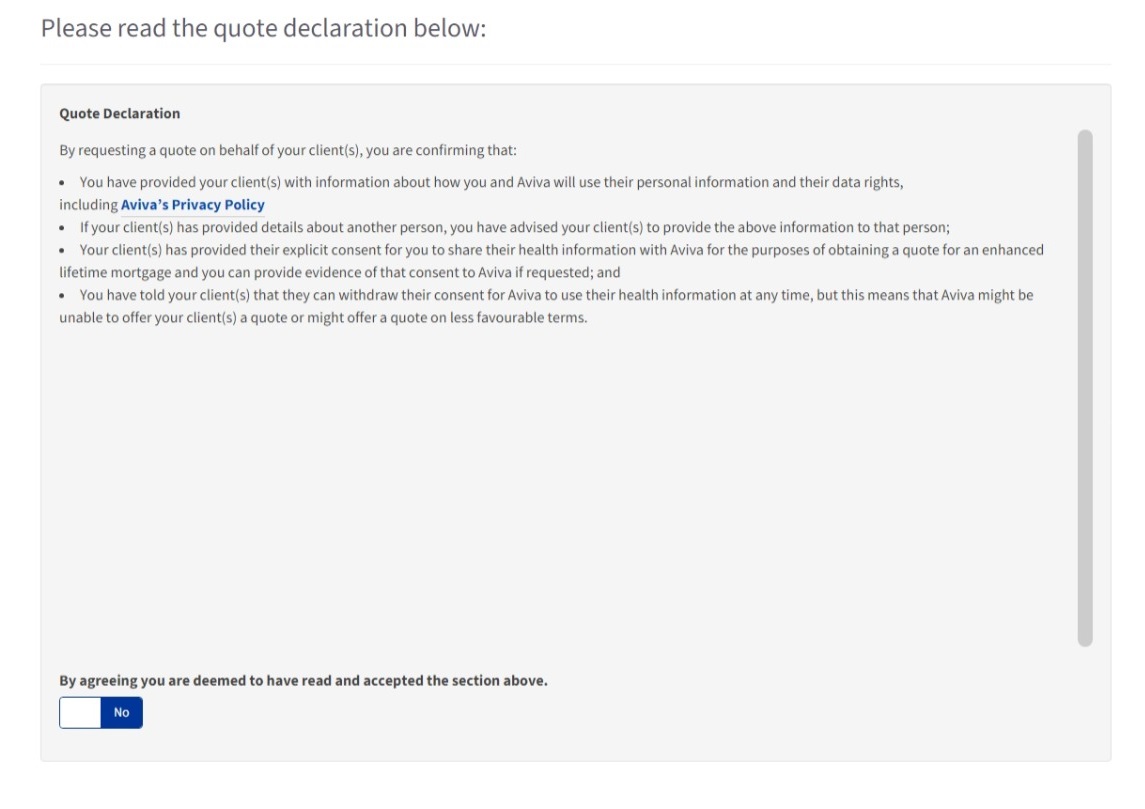This image is a screenshot of a form. The background is entirely white with dark gray text. At the top left corner, the heading reads "Quote Declaration" in black. Below this heading, the text instructs, "Please read the quote declaration below."

A large, gray form is presented in the center of the image. On the right side of this form, there is a vertical scrollbar, indicating that more content can be revealed by scrolling down if necessary. 

The main body of the form includes the following bullet points:

- You have provided your client with information about how you and Aviva will use their personal information and their data rights, including a link to Aviva's privacy policy.
- If your client has provided details about another person, you have advised your client to provide the above information to that person.
- Your client has provided their explicit consent for you to share their health information with Aviva for the purposes of obtaining a quote for an enhanced lifetime mortgage, and you can provide evidence of that consent to Aviva if requested.
- You have informed your client that they can withdraw their consent for Aviva to use their health information at any time.

In the bottom left corner, there is a toggle switch accompanied by the statement: "By agreeing, you are deemed to have read and accepted the section above." Currently, the toggle switch is set to "No" (displayed in gray). To agree, the user must toggle it to the left, which will change the display to "Yes" and highlight the switch in green.